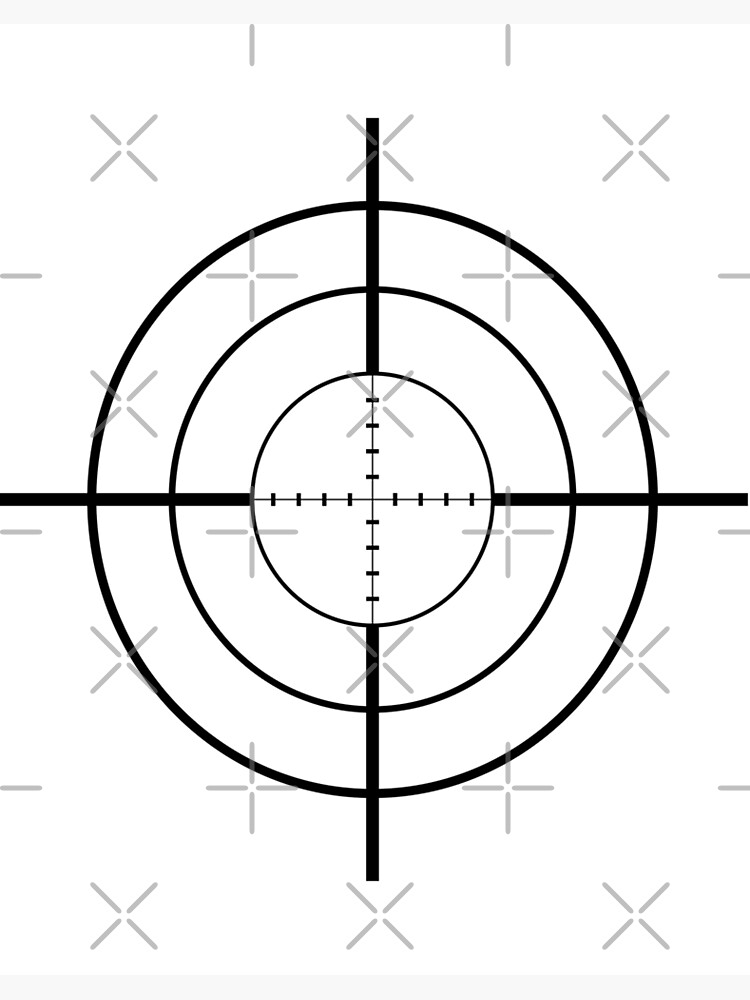The image depicts a detailed target or reticle design, reminiscent of a sniper scope crosshair or a bullseye used in target practice. Central to the design are three concentric black circles with a thin black cross intersecting at the center. This cross features a series of smaller black lines extending vertically and horizontally. Additionally, four thicker black lines emanate outward from the central circle, traversing through the second and third rings. The entire design is set against a white background, which is overlaid with a series of light gray, semi-transparent watermarks in the form of alternating crosses ('+') and X's. These watermarks partially cover the reticle but remain see-through, maintaining the visibility of the target design. Gray rectangles are also present at the top and bottom of the image, adding to the structured appearance.